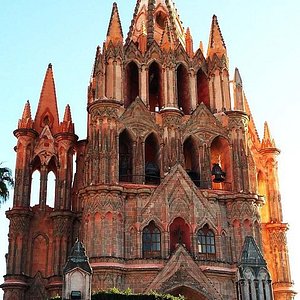This exterior photograph captures a grand, Gothic-era cathedral bathed in sunlight. Constructed from reddish-brown stone, the building exhibits masterfully done stonework featuring various geometrical shapes. The facade is adorned with tall archway formations and a multitude of cylindrical and conical spires reminiscent of a castle's turrets. The cathedral's imposing structure rises to at least three or four floors, culminating in elaborately adorned steeples that are rich in orange and red hues.

Standing out amidst the intricate architecture are several tall, pointed spires and windows that house bells. The complex design of the pillars, comprising multiple combined pillar-like shapes, adds to the grandeur of the building. The right side of the cathedral, illuminated by the morning sun, appears more yellowish compared to the left, which retains a darker tone due to the shadow.

In the background, a light blue sky fades horizontally to almost white, adding a serene atmosphere to the image. A tall palm tree on the left provides a tropical touch to the scene, while a light pole and some greenery can be seen at the bottom edge, further framing this impressive historical structure. Despite its beauty, the cathedral shows signs of wear, with grime and smog visible on its surfaces, hinting at its long-standing presence through the ages.